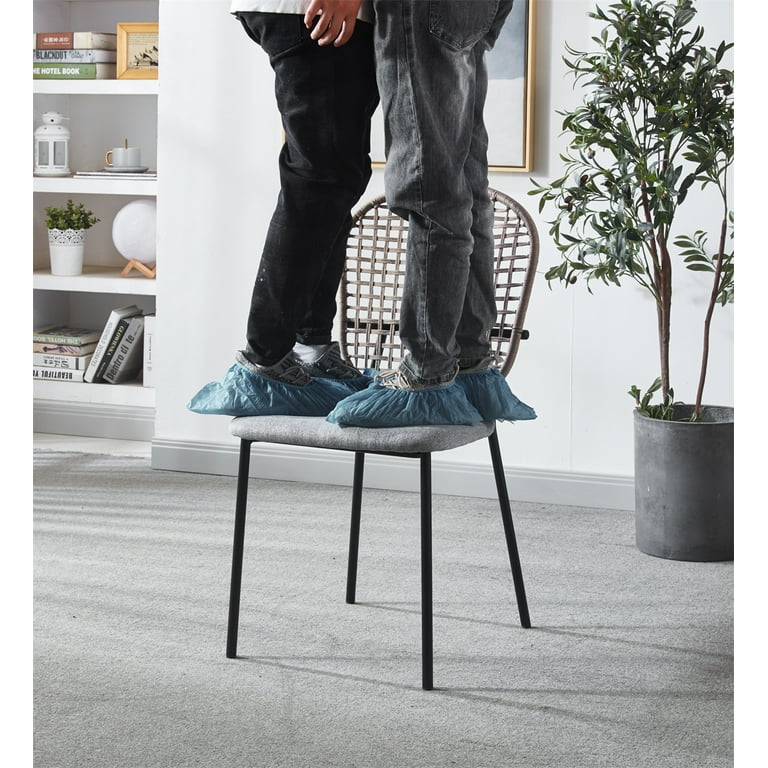In this indoor photograph taken in someone's home, a striking scene is captured. The room features white walls, with a noticeable recessed shelving unit that is filled with various items such as a framed picture, books, a mug, and a small plant. Dominating the room is a modern chair with skinny black metal legs, a dark gray cushion, and a light gray color scheme. The backrest is made of woven brown wicker. Standing atop the chair are two people, visible only from the torso down. Their shoes are covered with light blue protective shoe covers to prevent dirt from being tracked in. The individual on the right wears gray jeans and grayish-tan shoes, while the person on the left sports black jeans and similar colored shoes. The carpet beneath the chair is a matching light gray, contributing to the room's cohesive aesthetic. To the right side of the chair stands a large potted plant with lush green foliage, housed in a sizable gray pot, adding a touch of nature to the clean, minimalist space.